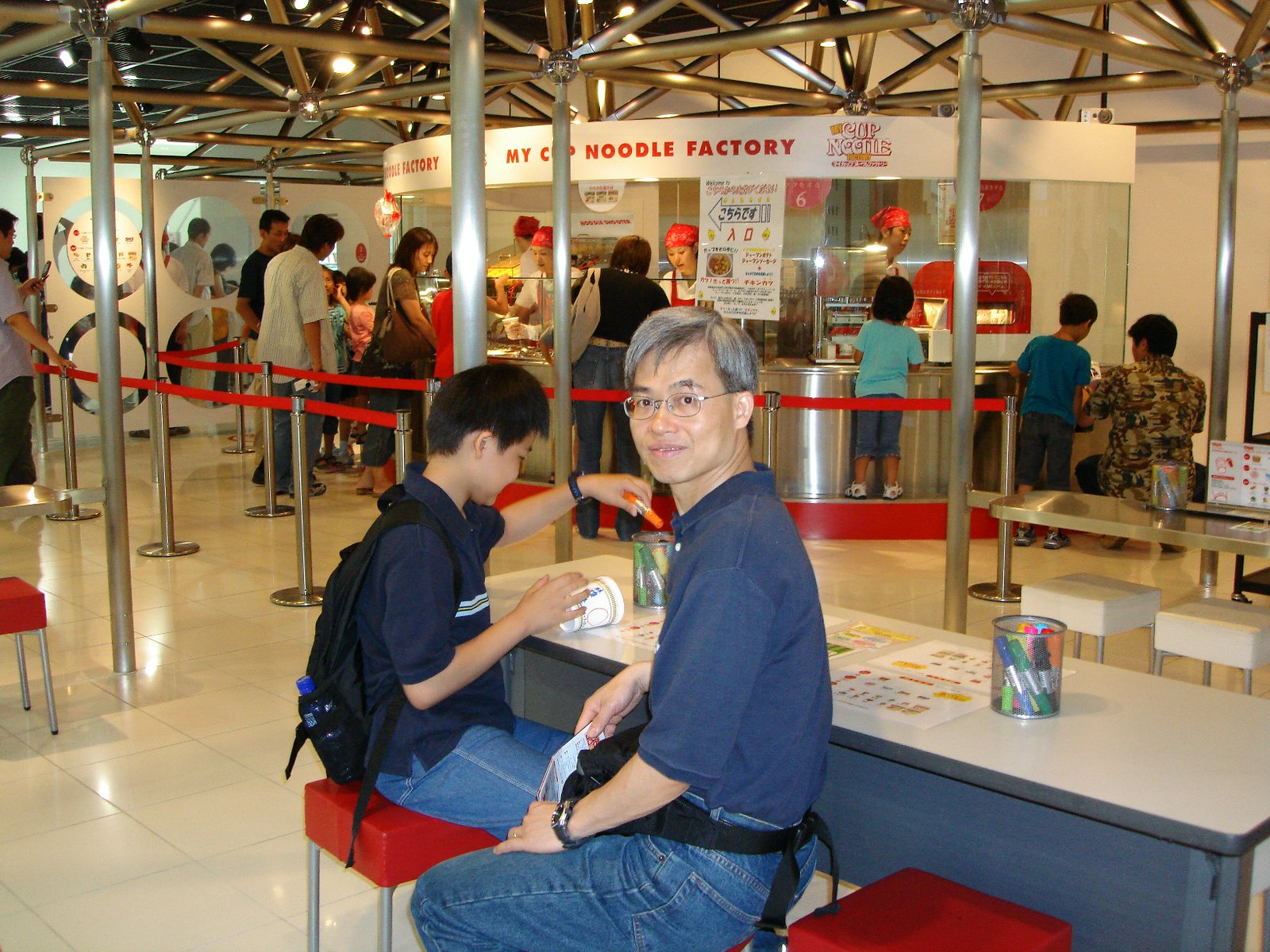In the bustling food court, a vibrant scene unfolds around the "My Cup Noodle Factory" kiosk prominently displayed in the background. The kiosk's sign features a stark white background with bold red capital lettering that catches the eye. A queue of eager patrons forms in front of the kiosk, corralled by orderly red stanchions as they await their turn to customize their cup noodles. 

In the middle foreground of the image, two individuals are seated at a low table accentuated by bright red stools. On the left, a young boy dressed in a dark polo shirt and with a backpack slung over his shoulders is absorbed in his own world, his face captured in a thoughtful right-side profile as he looks downward. Next to him, an older man with a full head of grey hair and glasses sits wearing a blue polo shirt. Their close proximity suggests a familial connection or close companionship, adding a warm, personal touch to the lively atmosphere of the food court.